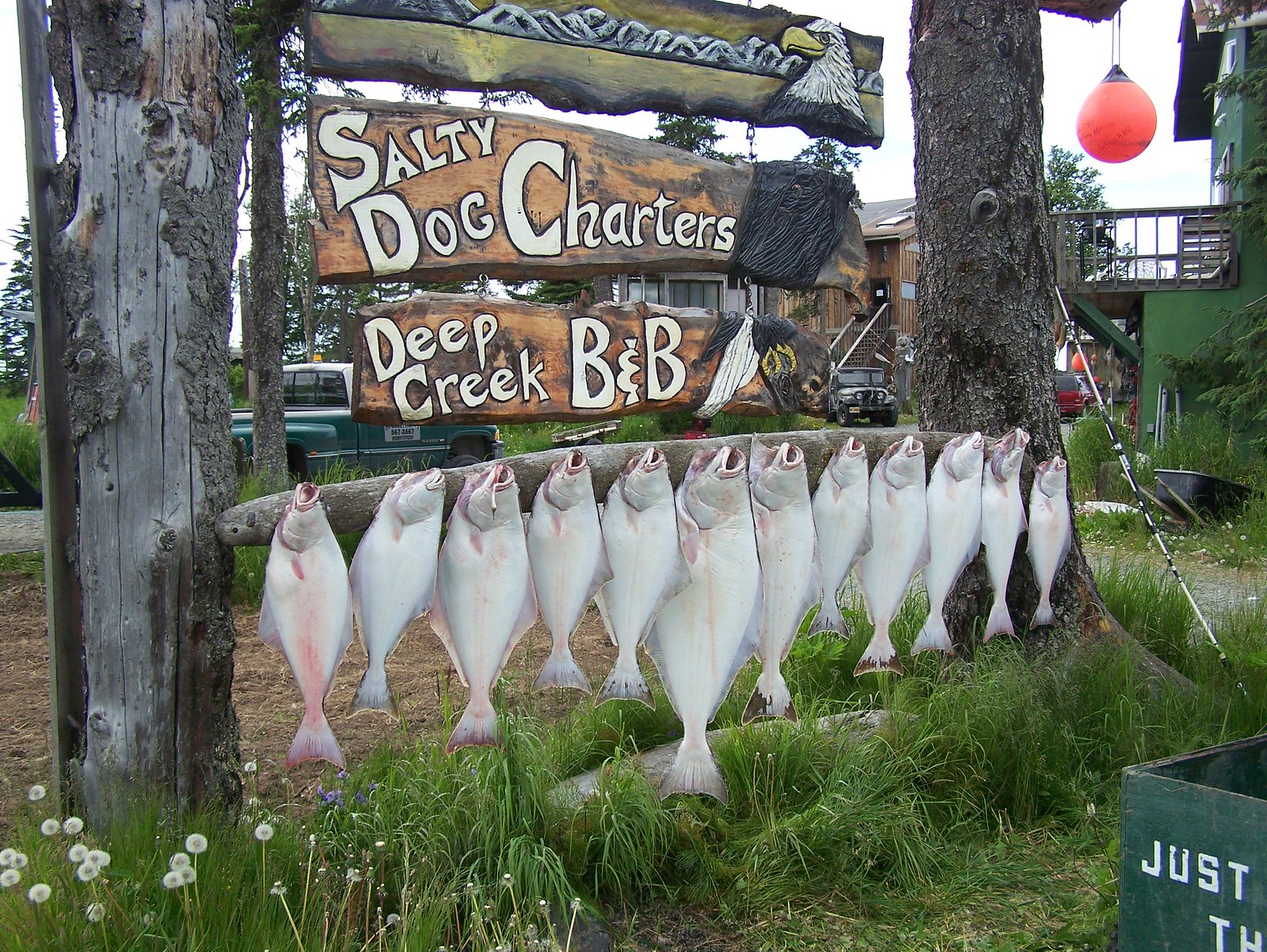The image depicts a vibrant, outdoor scene centered around a rustic, wooden signpost situated in a grassy dirt field. The signpost, adorned with playful, beach-themed designs, prominently displays two signs: "Salty Dog Charters" and "Deep Creek B&B". These signs are painted to evoke a fun, tropical ambiance and feature a pair of artificial fish hanging below them. An eagle painted in front of mountains crowns the signpost, enhancing the scenic aesthetic.

Positioned directly in the center of the image, the signpost is surrounded by a mix of natural and man-made elements. To the right, a roadway ascends into the scene, leading to several parked vehicles and a distant building. The sky forms the backdrop at the top of the image, adding to the midday outdoor ambiance. Several trees dot the landscape, further framing the scene. The colors present include a mix of green, white, yellow, pink, brown, and tan, contributing to the overall lively and picturesque setting.